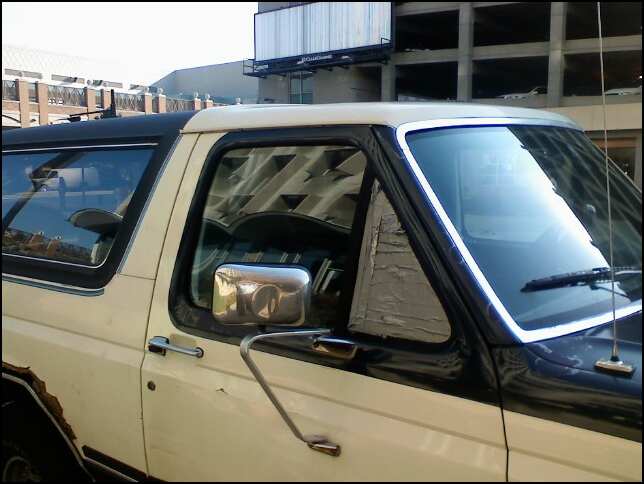This photograph, taken outdoors under a gray and hazy sky, captures a vintage 1980s vehicle, possibly a Jeep or a Bronco, though some describe it as a pickup truck with a shell. The vehicle is primarily white with distinct dark blue or black trim around the windows, windshield, and hood. Notable features include a silver mounting apparatus for a large side mirror, an antenna, and windshield wipers. The vent window on the passenger side is conspicuously covered with duct tape, and there's visible rust on the back fender. The truck's bed is topped with a black shell featuring large, shiny windows. The backdrop features a multi-level parking structure and a building with red brick columns and gray concrete slabs, alongside a blank white billboard. The close-up angle of the photo limits the view to the side and front of the vehicle, making the wheels mostly out of sight.